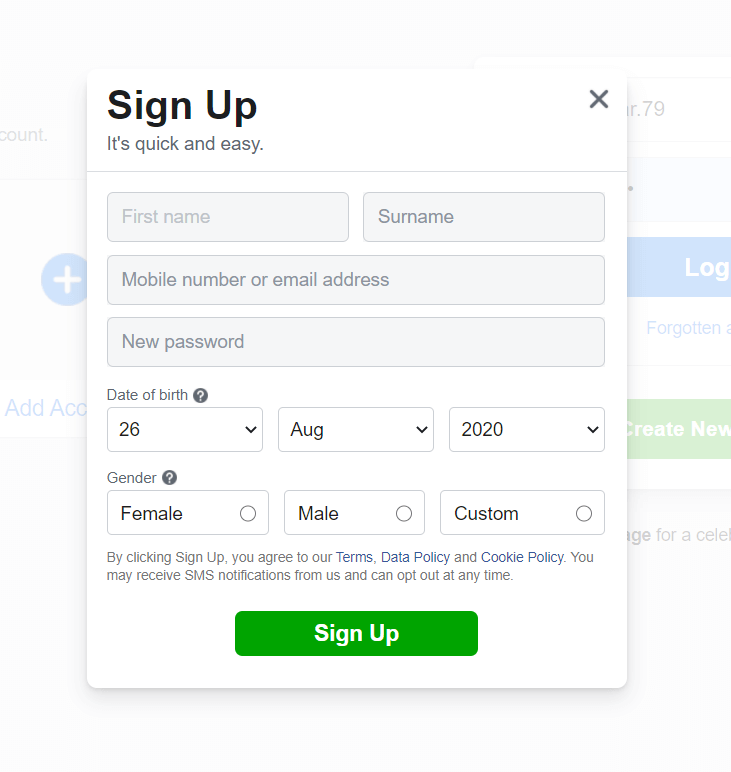A detailed screenshot of an online sign-up form. The primary focus is on a pop-up window prompting users to create a new account. The pop-up window dominates the image, obscuring parts of the background. The window features text that reads: "Sign up, it's quick and easy." Below this message are several input fields labeled as follows: "First name," "Surname," "Mobile number or email address," "New password," and "Date of Birth," which is pre-filled with "26 August 2020." Further down, there are gender selection options: "Female," "Male," and "Custom." At the bottom of the pop-up window, a green rectangle with white centered letters displays the text "Sign Up." Additional text indicates that by clicking "Sign Up," users agree to the terms, data policy, and cookie policy, and mentions the possibility of receiving SMS notifications with an option to opt out. The image is entirely textual, with no photographic elements or depictions of people, animals, plants, vehicles, or buildings.